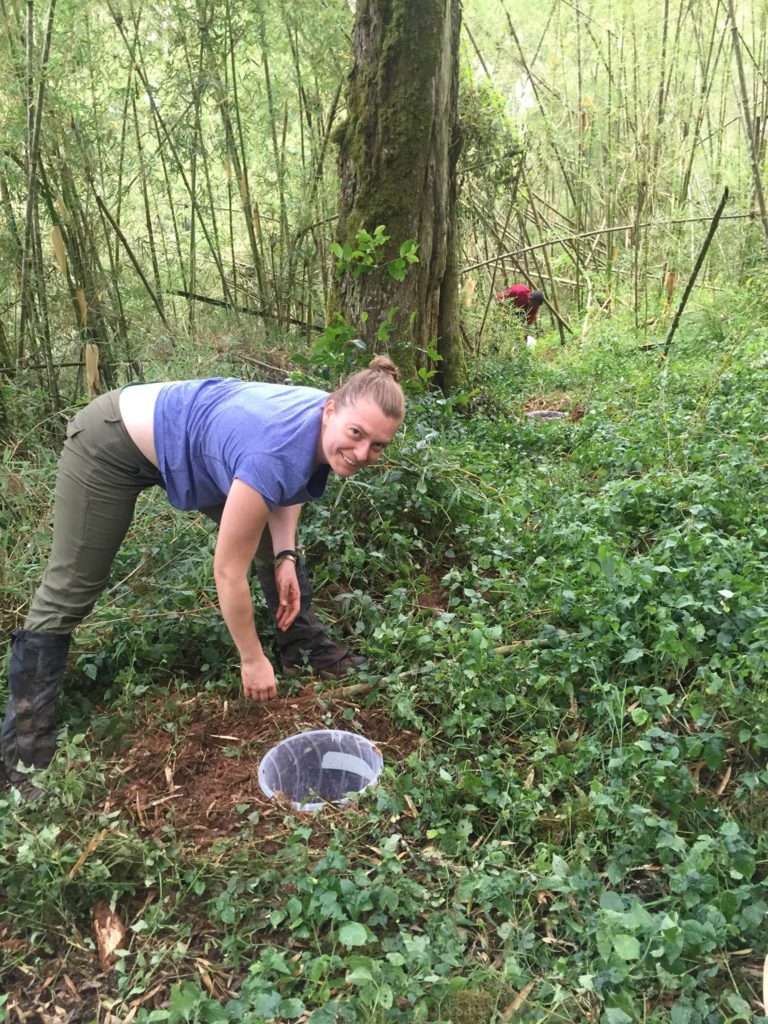In this detailed image, a woman is partially hunched over in a forest clearing, her light brown hair pulled back into a bun. She is dressed in a blue t-shirt, green pants, and black boots. Her left arm sports a watch and a bracelet. Positioned next to her is a long object resembling a walking stick or spear. The ground around her is covered in leaves, weeds, and underbrush, with a transparent plastic bucket embedded in the soil from a recently dug hole. She appears to be reaching into the bucket while smiling at the camera. Behind her, a forested area with a mix of thin trees and one notably thick tree partially obstructs the sky. In the background, there is another person in a red shirt carrying a similar bucket, indicating they might be setting up traps or collecting samples.